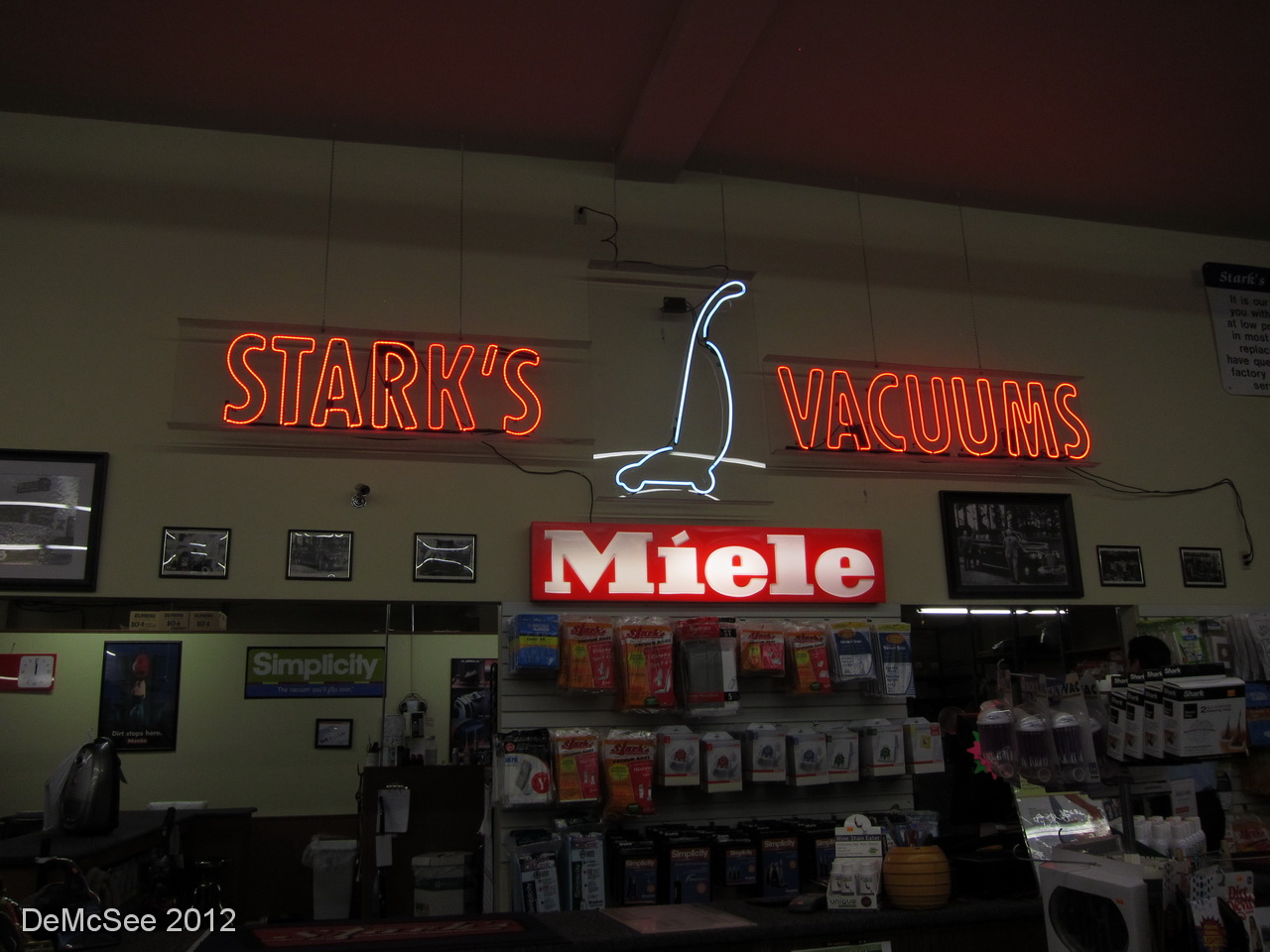This photograph captures a dimly lit interior of a store, showcasing a striking neon sign at the top. The sign reads "STARK'S VACUUMS" in bold, neon red letters, flanking a neon blue silhouette of a vacuum cleaner. Just below, the brand name "Miele" is displayed prominently in white font on a red rectangular background. The foreground includes shelving units adorned with various vacuum parts and accessories. The backdrop features a high, yellow-painted wall, adorned with framed photos near the ceiling. Lower on the wall, more shelving and framed signs are visible. In the bottom left corner of the image, the text "DEM CSEE 2012" is subtly written in white.